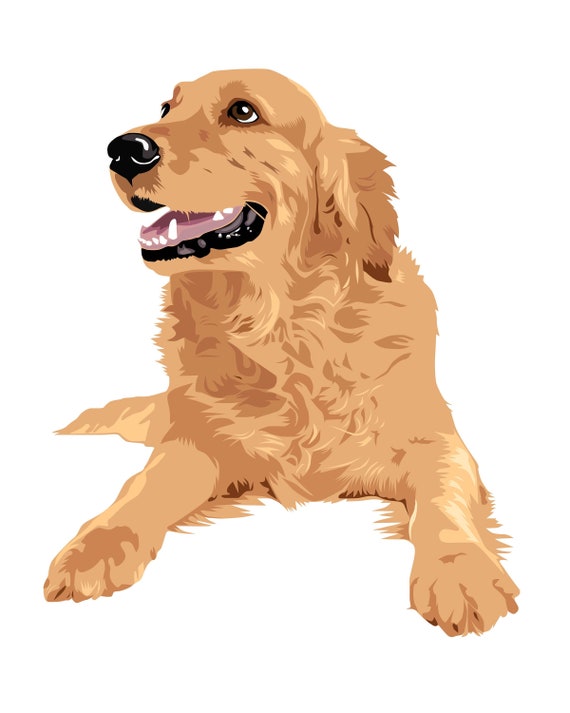This image is a detailed digital painting of a Golden Retriever dog lying down, with a white background. The Golden Retriever has light tan fur with a mix of blonde and slightly darker streaks, especially noticeable on its ears. Its mouth is open, revealing some black inside and its teeth, as though it is begging or expecting a treat. The dog’s head is turned slightly to the left, and it has expressive brown eyes that look a bit sad or longing. Its black nose stands out against its fur. The dog’s front paws are stretched out in front of it, and its tail extends behind it to the left. This realistic and intricately detailed CGI-like artwork captures the charming and cute essence of the dog, highlighting its furry texture and nuanced coloring.